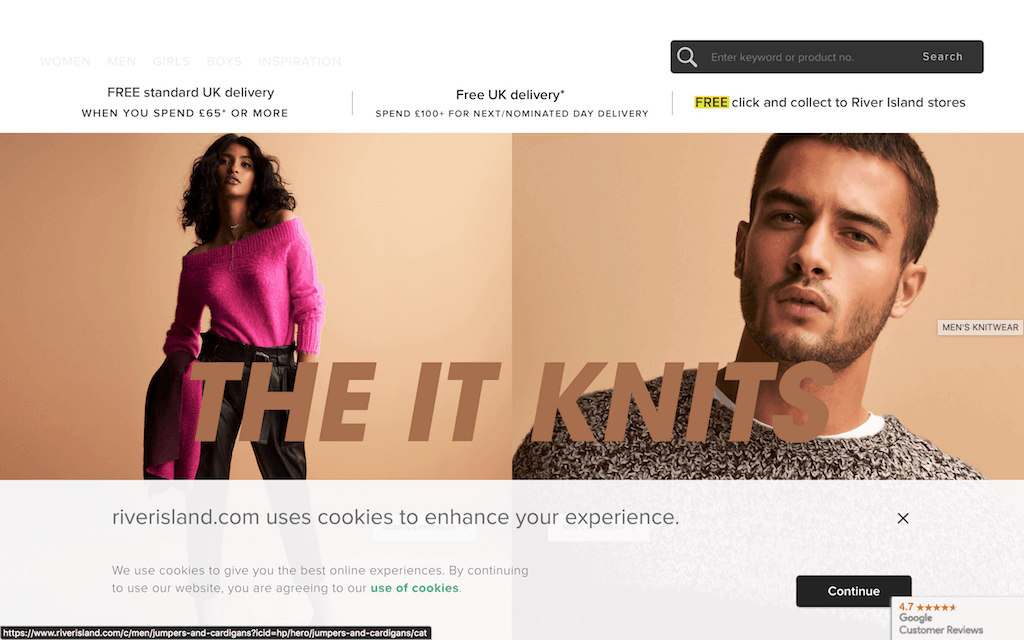This is a detailed caption for the website RiverIsland.com:

"The homepage of RiverIsland.com features a clean and user-friendly design. At the top, visitors can find navigation buttons for 'Women,' 'Men,' 'Girls,' 'Boys,' and 'Inspiration' tabs. Adjacent to these tabs on the right is a convenient search bar, allowing users to quickly access specific items across the site. 

Just below the navigation tabs, to the left, there's an announcement banner offering 'Free Standard UK Delivery' on purchases over €65. Adjacent to this, it highlights 'Free UK Delivery' with an option for 'Next/Nominated Day Delivery' on spending €100 or more. To the far right of this banner, a special promotion for 'Free Click & Collect to River Island Stores' is prominently displayed with the word 'Free' highlighted in vibrant yellow.

Beneath this banner, the main section showcases striking images of professional models. On the left, a woman dressed in a chic magenta sweater and white faux leather pants poses confidently, though the text overlay partially obscures her outfit. To the right of her, a young, brown-skinned female model with brown hair stands elegantly. Further right still, a male model with a chiseled jawline, light beard, brown hair, and brown eyes sports a knitted pullover sweater. The text beside him reads 'Men’s Knitwear,' and spans across both the female and male models' images with the tagline 'The End Knits' in a rich brown font.

The bottom section includes a notification about the use of cookies for an enhanced browsing experience, which users can choose to close. Additionally, there's a 'Continue' button and an impressive rating of 4.7 stars from Google customer reviews. This engaging layout and array of options await visitors at RiverIsland.com."